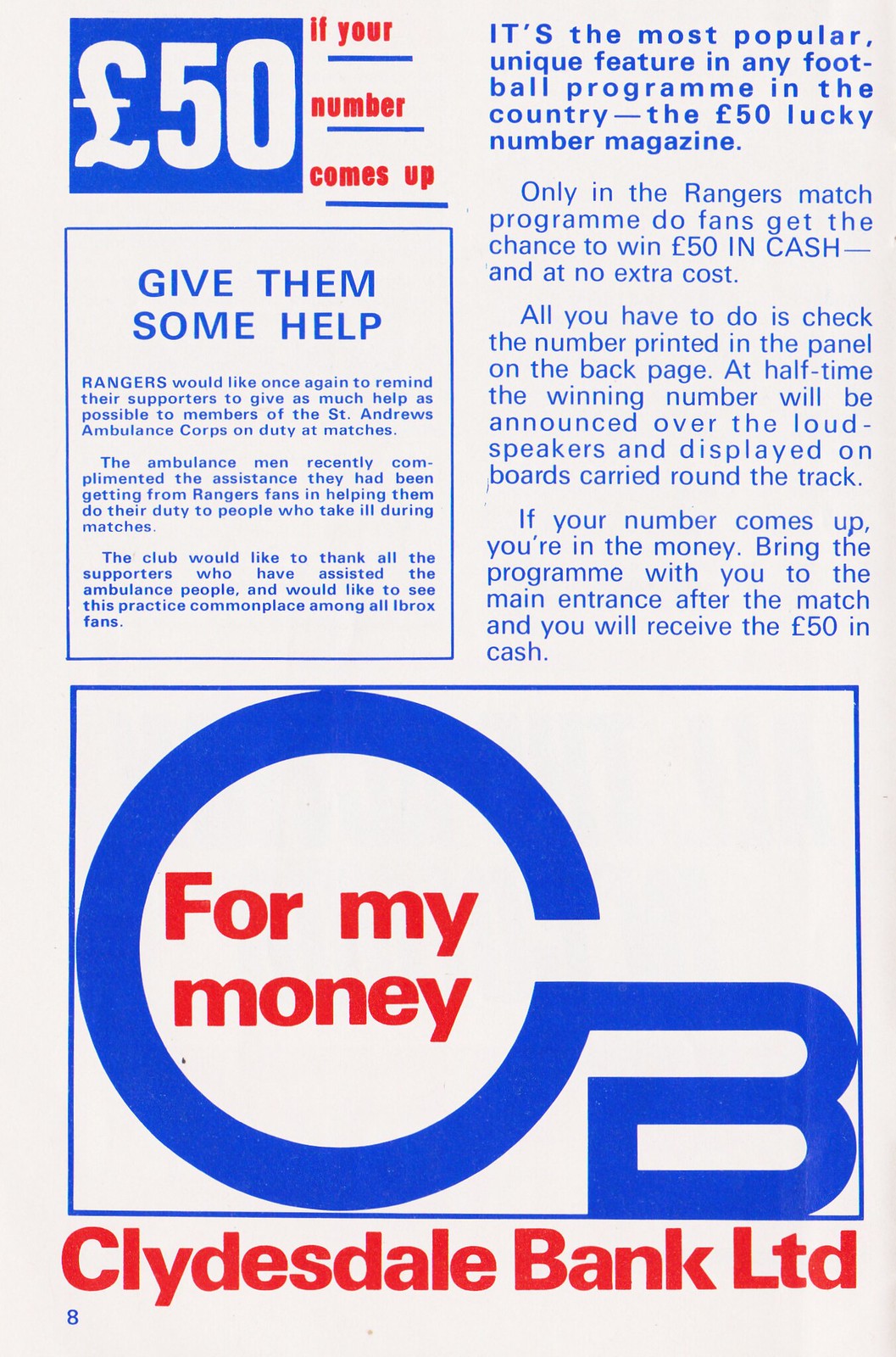This image is an advertisement featuring elements from a football magazine and likely promoting a bank. At the top left, a bright blue rectangle displays "L50" in white text, next to bold red text saying "if your number comes up," all underlined in blue. To the right, it announces the promotion as "the most popular and unique feature in any football program in the country," referring to the "L50 Lucky Number magazine." This promotion, exclusive to the Rangers match program, offers fans the chance to win L50 in cash at no extra cost by checking the number on the back page of the program. At halftime, the winning number is announced over loudspeakers and displayed on boards around the track. Winners can claim their prize by bringing the program to the main entrance after the match. A box at the left titled "Give them some help" reminds Rangers supporters to assist the St. Andrews Ambulance Corps during matches, thanking fans for their ongoing support and encouraging continued assistance. At the bottom, a large blue rectangle features a logo with a stylized "C" and a "B," enclosing the red text "For my money." Below the logo, in bold red letters, it says "Clydesdale Bank Limited."